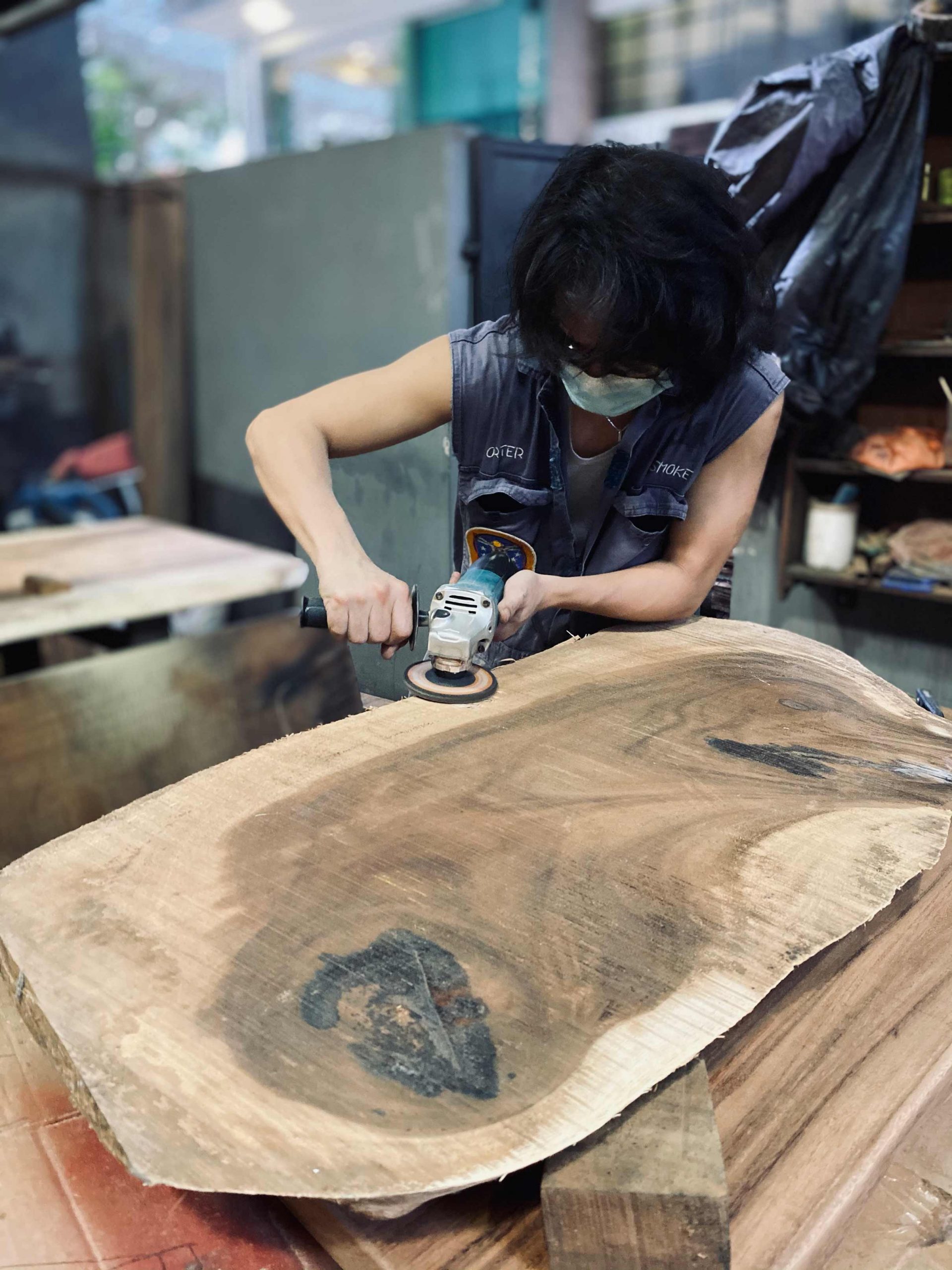The image depicts a focused woodworker in a concrete workshop, sanding a large, irregularly shaped piece of wood resting on a robust wooden workbench. The woodworker, a man with short black hair and donned in a blue sleeveless vest with white lettering and two large filled pockets, manages a motorized hand sander with both hands. His left elbow is propped on the wood, illustrating the intensity and control of his sanding technique. He also wears a mask and safety glasses, highlighting his attention to safety. The large piece of wood, likely freshly cut from a tree and featuring dark and black knots, bears signs of previous sanding with smoother edges. Behind the woodworker, the workshop reveals another workbench, various wooden slabs, shelves cluttered with random objects, a cabinet housing tools, and a protective curtain. The area appears slightly blurred, focusing on the diligent effort of the woodworker in the foreground.